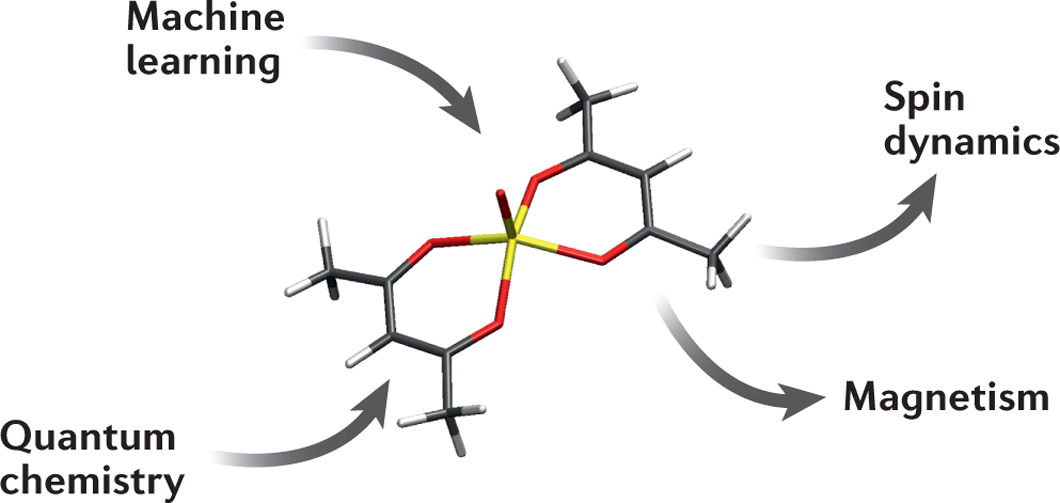The image displays a detailed 3D-rendered diagram of a chemical structure, composed of various colored elements and annotated to represent a flowchart. At the core, the structure features two benzene-like rings with interconnected black, white, red, and yellow components, arranged symmetrically. Grey tubes connecting black segments are positioned in the upper right, while similar black and silver connections are found in the bottom left. The middle section showcases red and yellow accents crossing the diagram.

Annotations in capital letters, except for certain words, label different parts of the diagram: "MACHINE LEARNING" is indicated at the top left, "SPIN DYNAMICS" at the top right, "MAGNETISM" at the bottom right, and "QUANTUM CHEMISTRY" at the bottom left. Arrows highlight the connections between these terms and the molecular structure: arrows leading to the structure denote "MACHINE LEARNING" and "QUANTUM CHEMISTRY," while arrows pointing outward indicate "SPIN DYNAMICS" and "MAGNETISM."

The detailed black lettering and gradient arrows from light gray to black add depth to the diagram, illustrating the complex relationships between the concepts in a visually sophisticated manner.